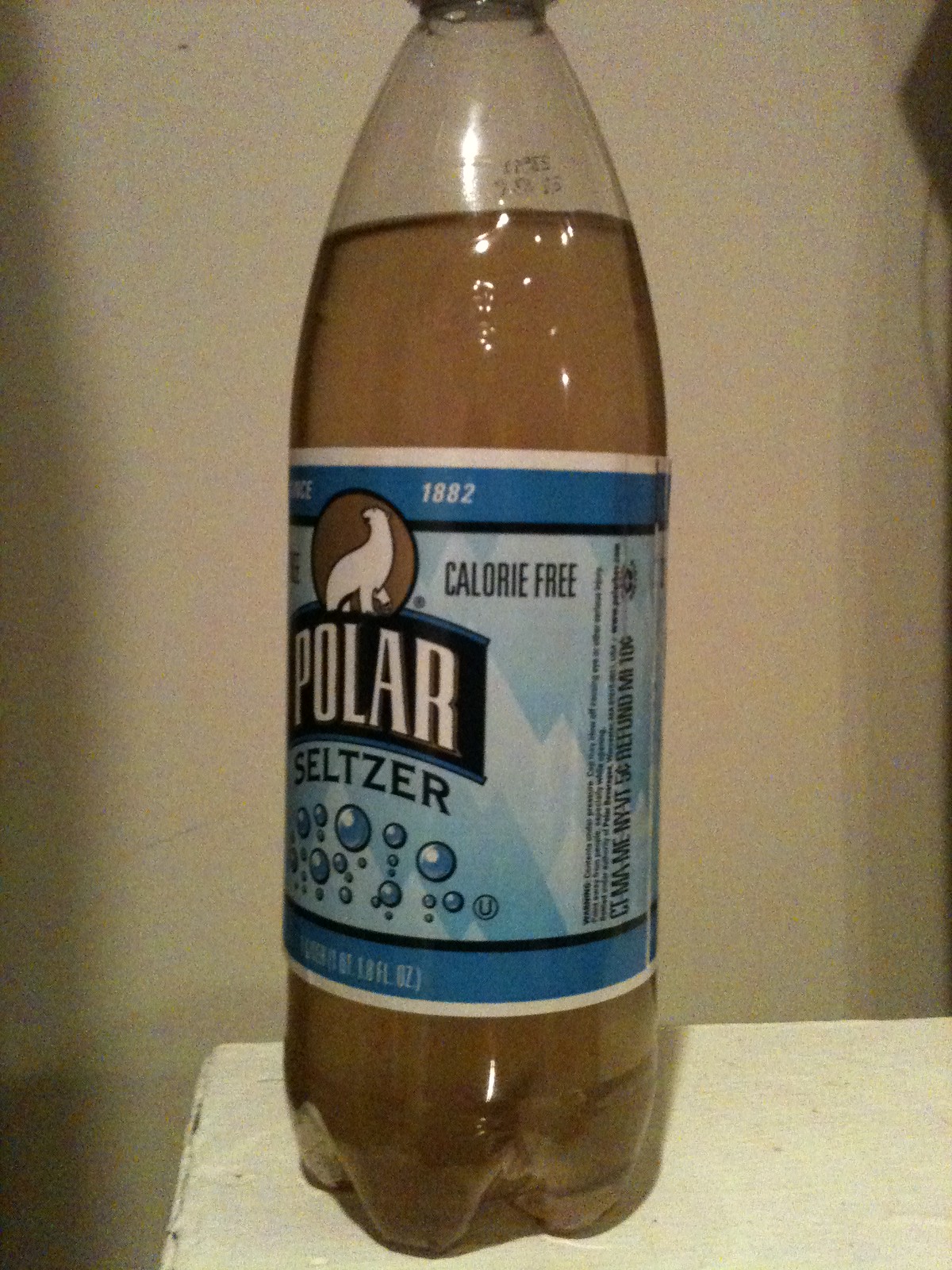This photograph showcases a plastic bottle of Polar Seltzer, positioned on the corner of a white wooden table with visible wood grain and signs of wear. The bottle is slightly turned to the right, revealing most of its label. The label features the words "Polar Seltzer" prominently in white text on a dark blue background with lighter blue accents. Above "Polar" is the date "1882," and below are decorative blue bubbles. The label also includes a white drawing of a seal within a golden circle. The bottle is filled with a clearish brown liquid, casting shadows on the left and right due to a light source above. An off-white wall serves as the backdrop, adding to the image's overall composition. The photograph appears slightly out of focus, but the details of the label, including the calorie-free claim, are still discernible.